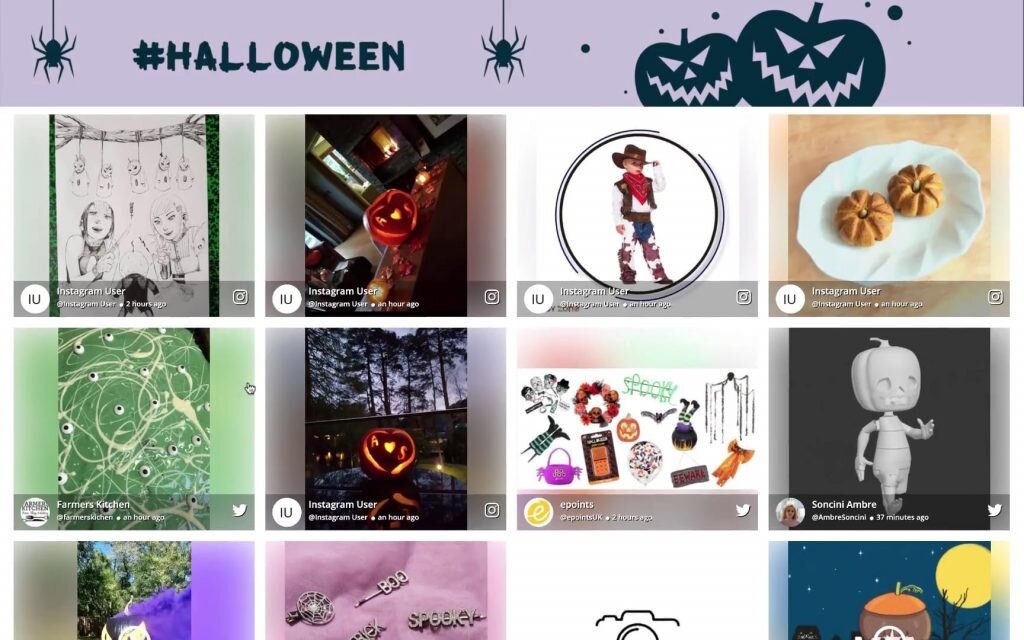The image depicts a shopping website with a festive Halloween theme. At the top, there's a light purple banner that prominently displays the hashtag "#Halloween" in black text. On the far left corner of the banner, a cartoon spider hangs down, adding a playful touch. Two more spiders and a couple of cartoon-styled pumpkin silhouettes are scattered across the banner, enhancing the spooky vibe.

Below the banner, the main content area consists of three rows, each with four images arranged horizontally. These images appear to be screenshots of social media posts, with each one having the respective Instagram or Twitter icon in the corner, indicating the source platform. 

In the top row, the far-right image stands out with a photograph of two small, real pumpkins. They are placed on a white decorative plate set on a table, embodying a simple yet elegant Halloween decoration idea.